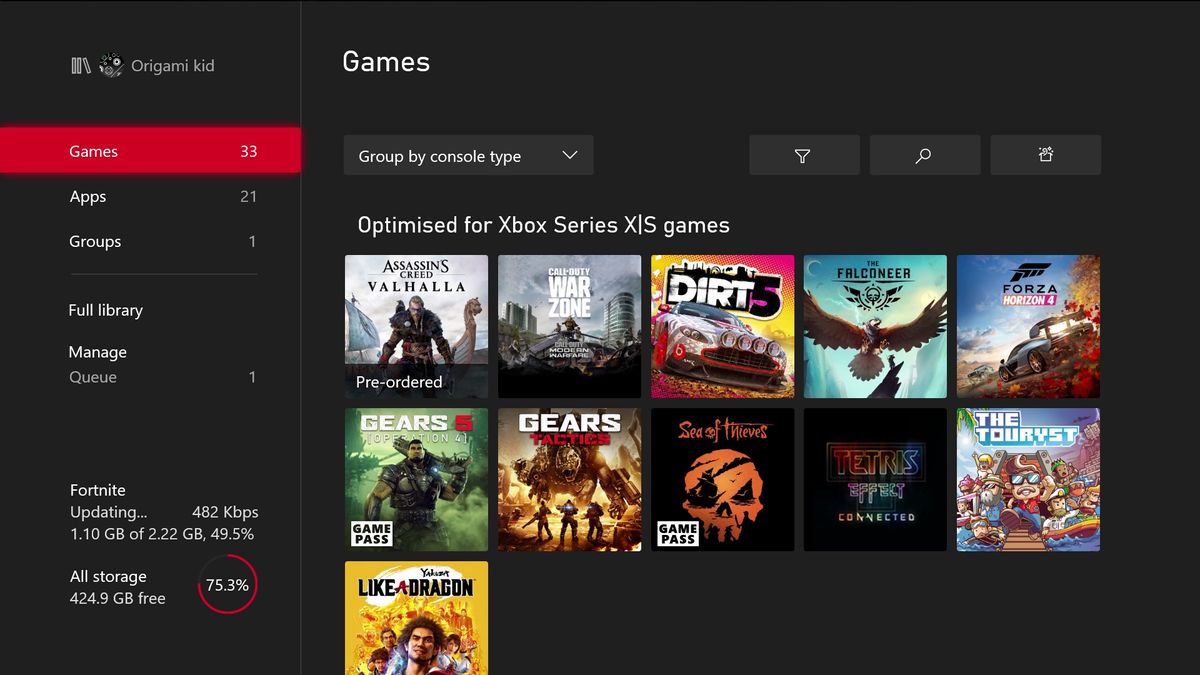The image showcases a rectangular interface with its long side orientated horizontally. The interface is predominantly black and divided into two main sections: a column on the left, occupying roughly a quarter to a third of the image, and a larger main body on the right.

### Left Column:
At the top of the column, there is a label that reads "Origami Kid" accompanied by several symbols to the left. Below it, there's a red rectangular box with white text displaying "Games 33." Further down, another set of white text reads "Apps 21," "Groups 1," "Full Library," and "Manage Queue 1." At the bottom of this column, an update status for "Fortnite" is displayed, showing "Fortnite updating... 482 kbps." Below that, the progress is detailed as "1.10 gigabytes of 2.22 gigabytes, 49.5%." Additionally, there is a storage report stating "All Storage 424.9 gigabytes free" accompanied by a red progress circle that is 75.3% complete, indicating the storage usage.

### Right Main Body:
At the top of the main body section, the word "Games" is prominently displayed. Underneath is an option labeled "Group by console type" featuring a drop-down arrow next to it. The interface also includes three buttons resembling a sound icon, a search icon, and a trash bin icon. Towards the bottom, a label specifies, "Optimize for Xbox Series X|S Games," indicating the type of games displayed or optimized within this section.

Overall, the image appears to be a user interface likely designed for a gaming console or platform, providing detailed information on games, updates, storage, and organizational options.